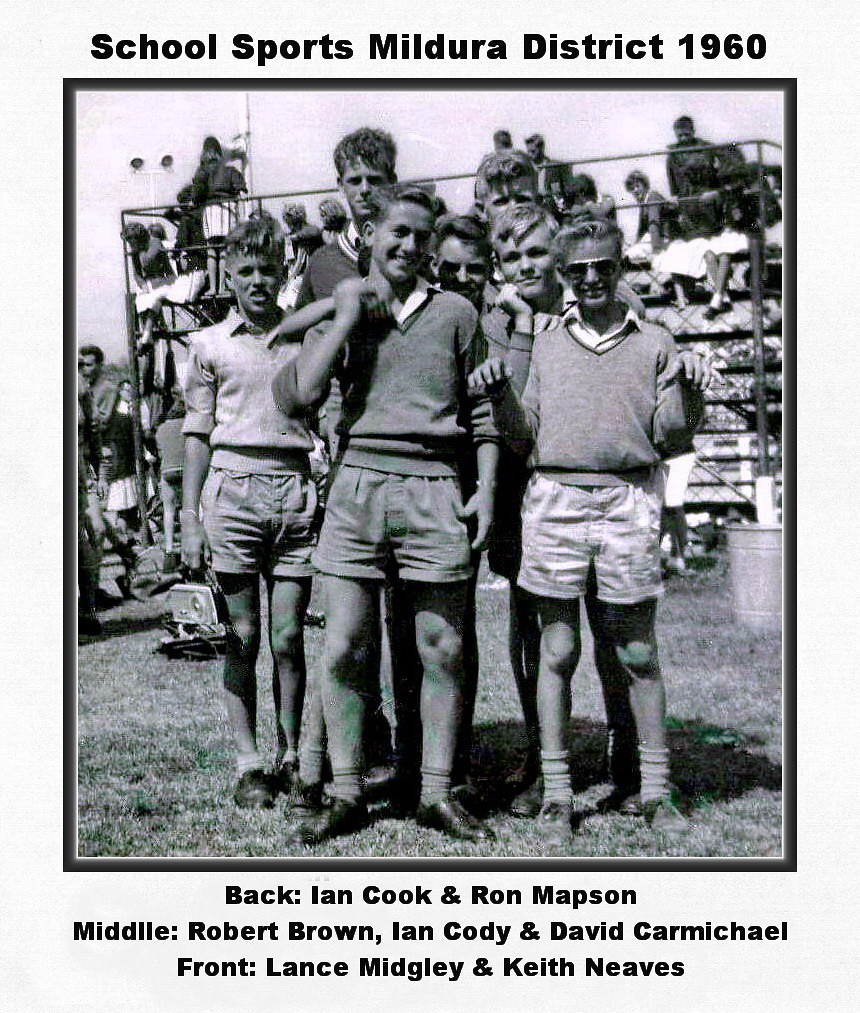The image is a black and white photograph from the early 1960s, framed by a light gray border with a thinner dark gray inner border. At the top of the border, the text reads "School Sports, Mildura District, 1960," and below the photograph are the names "Back: Ian Cook and Ron Mapson. Middle: Robert Brown, Ian Cody, and David Carmichael. Front: Lance Midgley and Keith Neves." The photograph captures seven young men posing in a grassy field with bleachers filled with students in the background. The students on the bleachers are mostly turned around, looking towards the camera, some appearing to be goofing around. The individuals in the photo are dressed casually in polo shirts and khaki shorts, with socks and not quite tennis shoes. Notably, the person on the far left wears a button-up shirt with a sweater vest and short pants, holding an old-fashioned silver radio. The person on the far right is wearing aviator sunglasses. The photo exudes a nostalgic feel, characteristic of the 1960s school sports era.